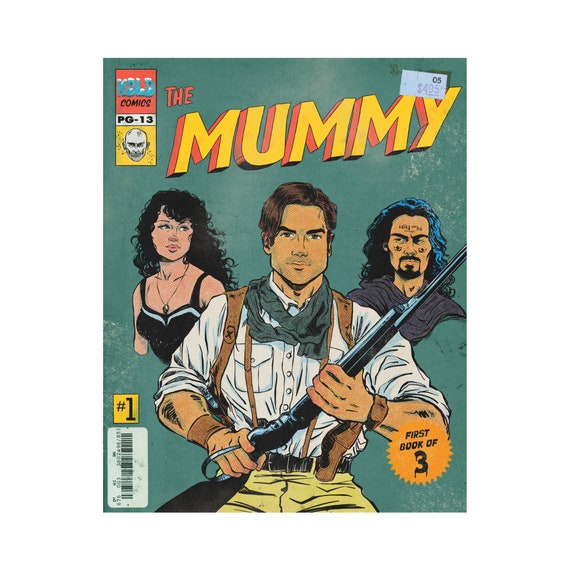This comic book cover is rectangular and about two inches wide by three inches high, featuring a greenish-blue background. At the top left corner is a sectioned orange square with blue text that reads "Cold Comics," a white rectangle labeled "PG-13," and a yellow square with an image of a bald man's head. The title "The Mummy" is prominently placed at the top center, with the words "The" in red and "Mummy" in large yellow letters outlined in red. On the top right corner, a blue rectangular sticker displays the price as $4.95. 

Central to the cover is a detailed drawing of Brendan Fraser's character, dressed in a white shirt, wearing a watch and an armband on his right arm, and holding a lever-action rifle, suggesting an adventurous, possibly jungle or archaeological setting. Behind his left shoulder is Rachel Weisz's character, depicted in a light blue and black halter top, wearing a necklace and looking to the right. Over his right shoulder is an ominous figure with dark black, blue-hued hair and a goatee, resembling a villain. 

In the bottom left corner, there is a small yellow square with a large number "1," positioned above a white rectangle that contains a barcode with black lines. The bottom right corner displays a gold circle with black text reading "First Book of Three." This cover art not only defines its genre and characters but also sets a tone of adventure and mystery, enticing readers to dive into the story.